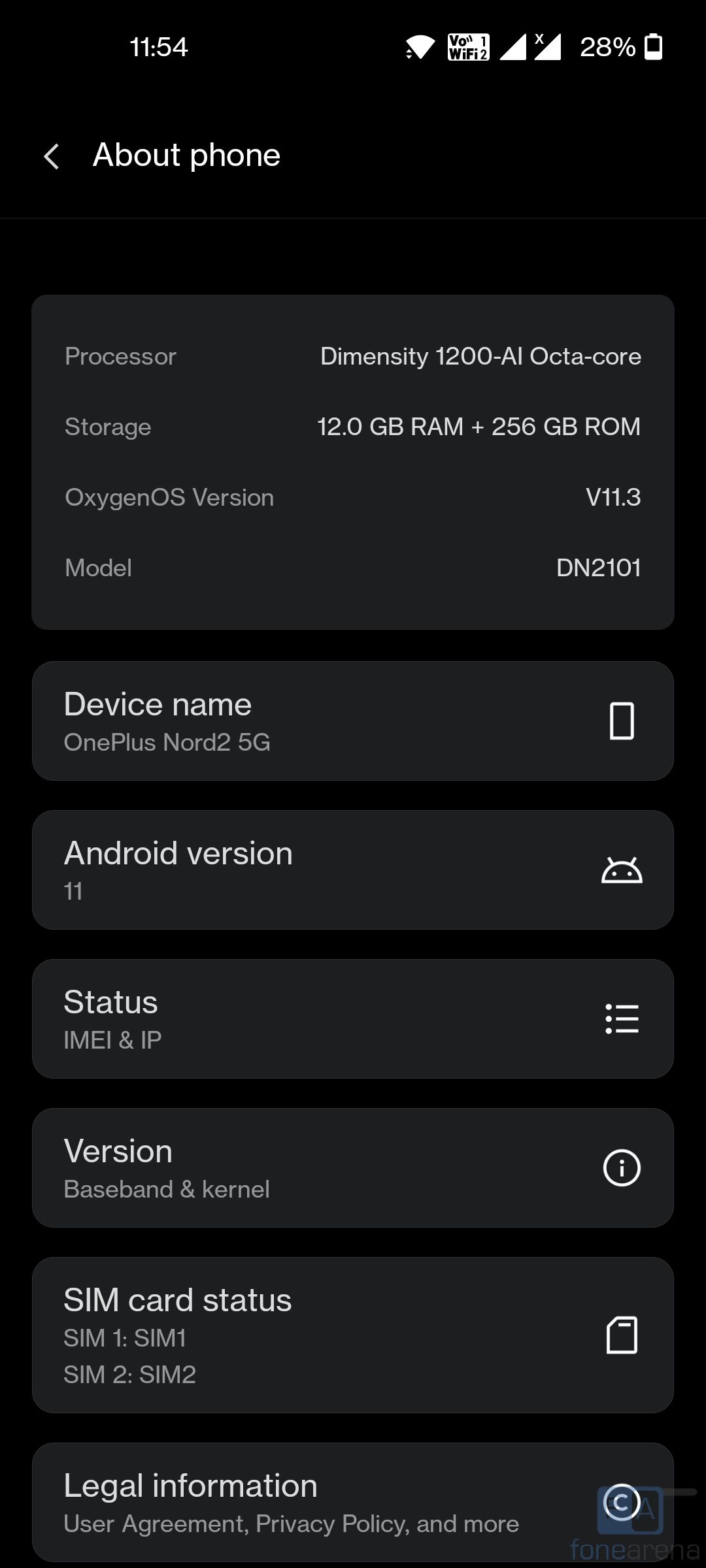The image is a screenshot taken on a mobile device, primarily featuring a monochromatic palette consisting of black, gray, and white tones. At the top of the screen, the time is displayed as 11:54, along with a fully filled Wi-Fi signal icon, carrier signal strength, and a battery life indicator showing 28% with the corresponding battery icon. An arrow pointing to the left is positioned at the very top, accompanied by the text "About Phone" in a white font.

Below this header, there is a prominent gray rectangular box containing detailed information about the device. The text within the box, presented in white, provides specifications such as the processor, listed as "Dimensity 1200 AI Octa-Core." The storage capacity is noted as "12.0 GB RAM and 256 GB ROM." Additionally, the device runs on "Oxygen OS version V11.3." The model number "DN2101" and the device name "OnePlus Nord 2 5G" are also specified. Further details include "Android version 11," alongside an illustration of the white Android mascot. The box also contains sections labeled "Status," "IMEI," and "IP," organized into three separate bars.